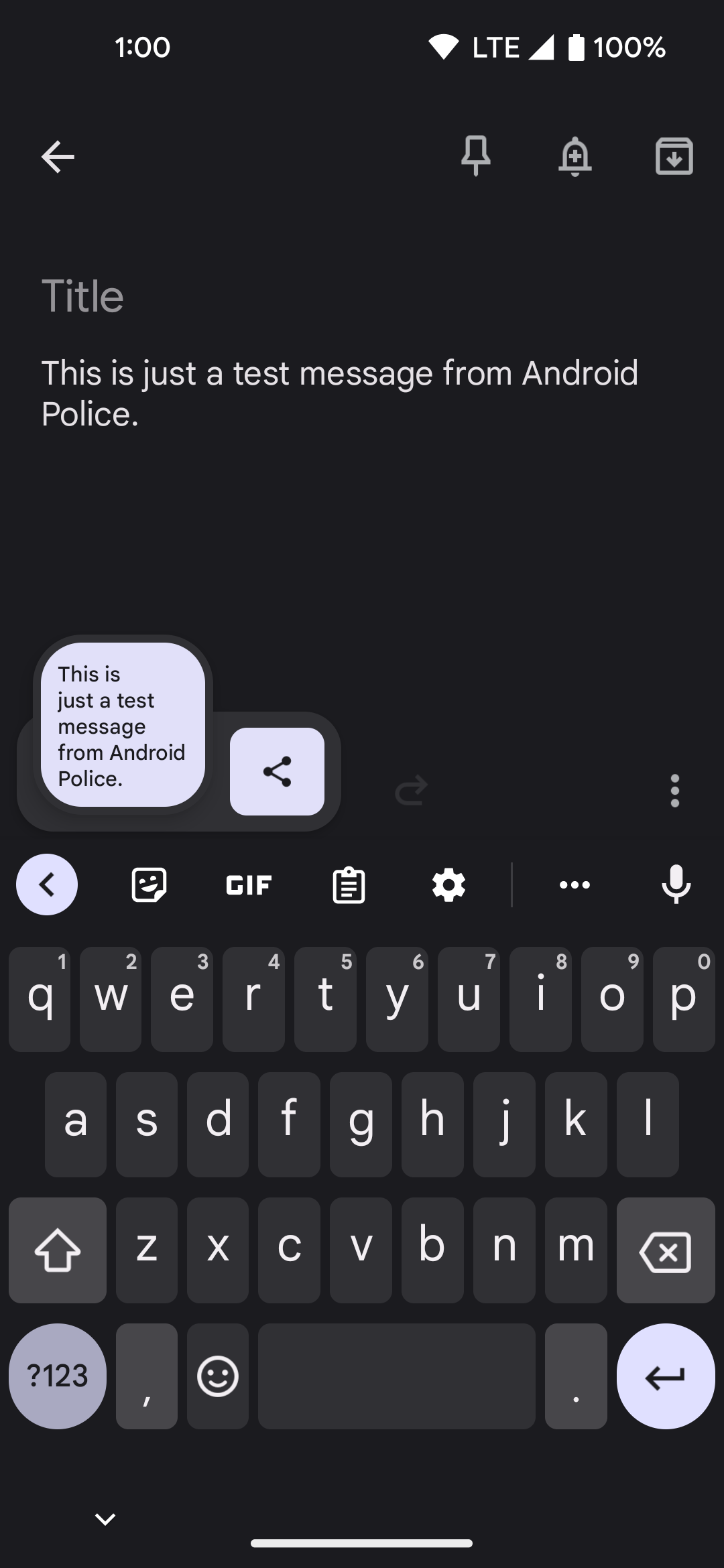### Caption for Image under the Category: Websites

The image shows a smartphone interface in dark mode, with a predominantly black background and white text. At the top of the screen, the time is displayed as 1 o'clock, though it is unclear whether it is AM or PM. The status bar indicates an active Wi-Fi connection, LTE network availability, full phone signal bars, and a battery at 100% charge.

Beneath the status bar, there's a navigation toolbar featuring a white back arrow, a thumbtack icon for pinning, a notification bell, and a download symbol. Following this toolbar, there's a text reading "Title," and just below it, a message stating "This is just a test message from Android Police." This message is repeated in a white square below, accompanied by a share icon.

The lower portion of the screen showcases the keyboard interface, including a back arrow, icons for stickers, GIF images, clipboard access, settings, more options (three dots), and a microphone for voice-to-text input. The on-screen keyboard layout is in standard QWERTY format, though it is not clear if swipe typing is enabled.